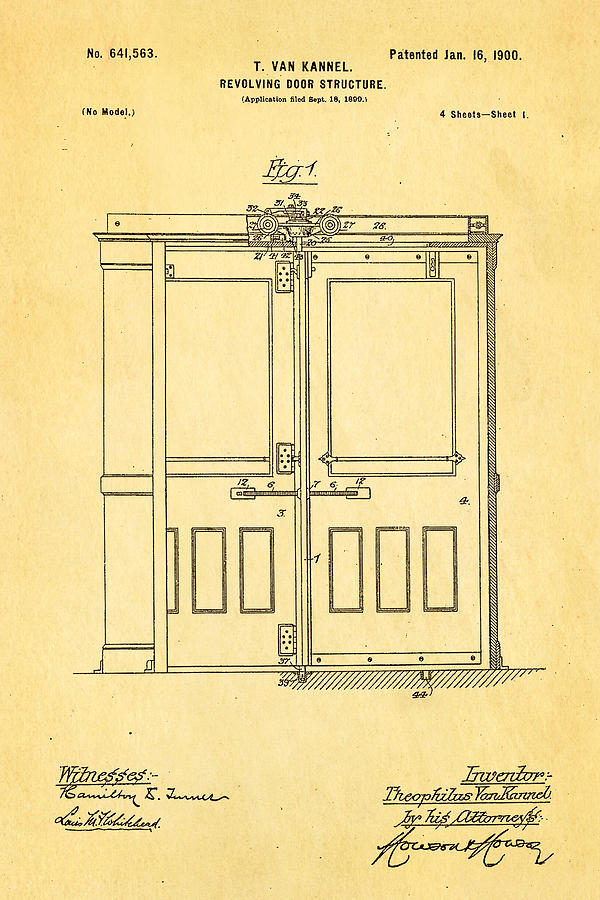This detailed drawing is a historic blueprint of a patented revolving door structure by inventor Theophilus van Kannel, dated January 16, 1900, and designated patent number 641,563. The blueprint, sketched in black ink on yellowed paper, depicts two door panels featuring large rectangles in the upper half and a series of small squares beneath. These panels are anchored by a central post and a side post on the right. Above the door, a technological mechanism, possibly gears, is indicated, likely illustrating the door's rotating function. The top of the document reads "T. van Kannel, revolving door structure," with an application date of September 18, 1899. Numbers label various parts throughout the detailed sketch. At the bottom, in handwriting, the blueprint bears signatures of witnesses on the left and indicates "Inventor Theophilus van Kannel by his attorney" on the right, both in cursive script.